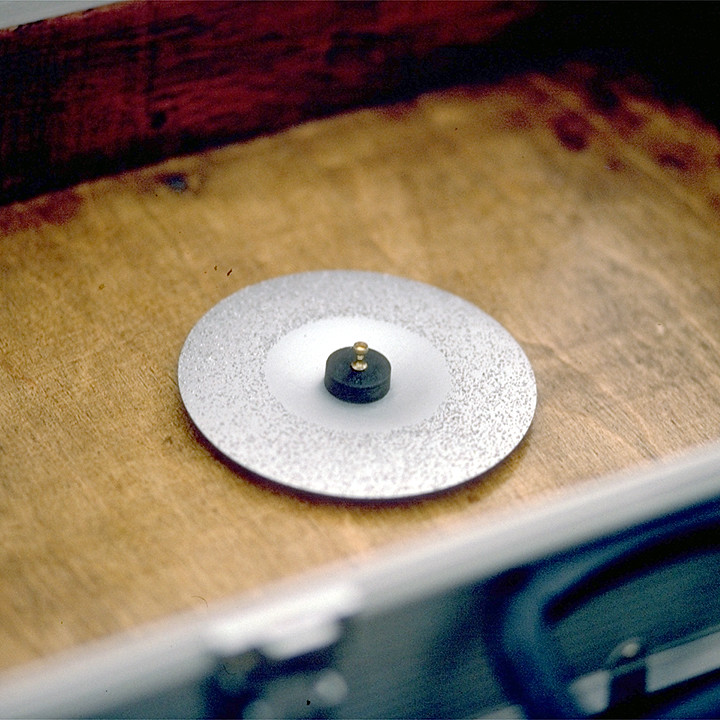The photograph displays a light wooden surface, heavily scratched and marred, with possible burn marks or brown discolorations along its edges. The surface is framed by a gray side featuring metal elements, including what appears to be a handle and locks reminiscent of a briefcase. Positioned prominently at the edge of this wooden surface is a round, silver metallic disc, distinguished by its pebbled edges and a smooth center. Embedded in the middle of this silver disc is a smaller, thicker black disc topped by a small, gold screw, resembling the head of a thumbtack. The backdrop showcases a darker wooden wall or shelf, enhancing the contrast between the light wood surface and its surroundings.